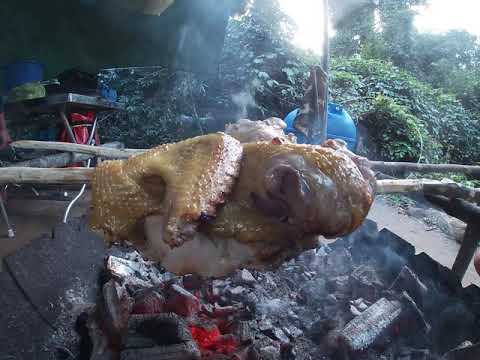In this vivid image, set within a dense, forested area that resembles a jungle, we observe a rustic outdoor cooking scene. The centerpiece of the photo is two skewered animals—potentially chickens or some other winged creatures—mounted on wooden sticks and being slowly cooked over an open flame and glowing red-hot coals. The skewers appear rotisserie-style, suggesting they can be rotated for even cooking. Adjacent to the coals is a second skewer with another animal, adding to the feast. 

The setting is marked by a backdrop of thick, verdant trees and shrubs. A wooden pole, adorned with a brown towel, stands out in the background, next to a blue water container that further emphasizes the makeshift nature of the campsite. To the left, partially obscured by foliage, is a table with a red object beneath it and a black pot resting on top, hinting at additional cooking activities. The entire scene is illuminated by what appears to be natural daylight, filtered through a cloudy sky, contributing to the rugged, untamed atmosphere of this primitive cookout.